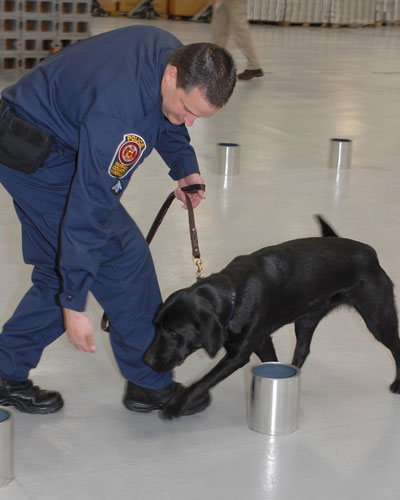In the photograph, a white man with short brown hair, clad in a blue uniform resembling a security or police jumpsuit with a distinguishing red and yellow patch on his right shoulder, is seen possibly training a young black Labrador. The man, donning black boots and a black fanny pack positioned to his side and back, is bending down, holding his right hand near the ground as the dog intently sniffs at it. His left hand holds a brown leather leash attached to the dog. The setting appears to be indoors, potentially an airport, given the expanse of white linoleum flooring. Scattered across the floor are various small containers, resembling silver metal cylinders or paint cans, indicating an early training phase for the dog, possibly for sniffing out illicit substances. In the background, cinder blocks and short posts can be seen, and a person in khaki pants walks away, further contextualizing the environment.